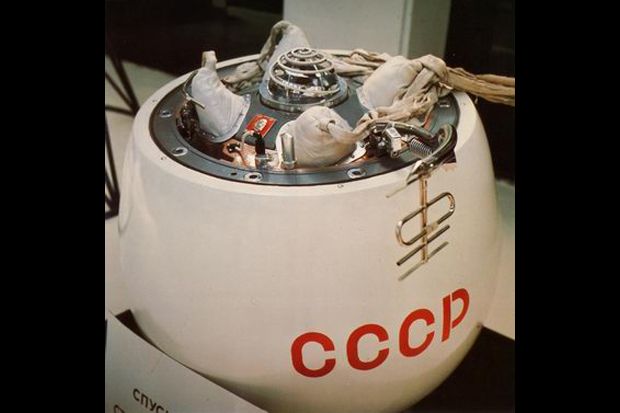This image showcases a cylindrical, white mechanical device resting on a white surface with a black background. The device appears to be made of ceramic material, giving it a smooth and polished appearance. The lower portion of the device prominently displays the bold red letters "CCCP," indicating its Soviet origin. A metal section covers the center, secured by multiple screws, and the top appears to have been removed or exposed, revealing a complex arrangement of metallic components and possible electronics. Surrounding a central circular metal piece on top are various cloth-like coverings draped over different items, alongside four small white structures evenly spaced at 90-degree intervals. Adding an intricate touch is a spiral metal element emerging from the center. The photograph is square, bordered thickly in black, and illuminated by what seems to be artificial light. In the lower-left corner, there's a white placard with unreadable brown Russian writing, adding to the intrigue of the scene.